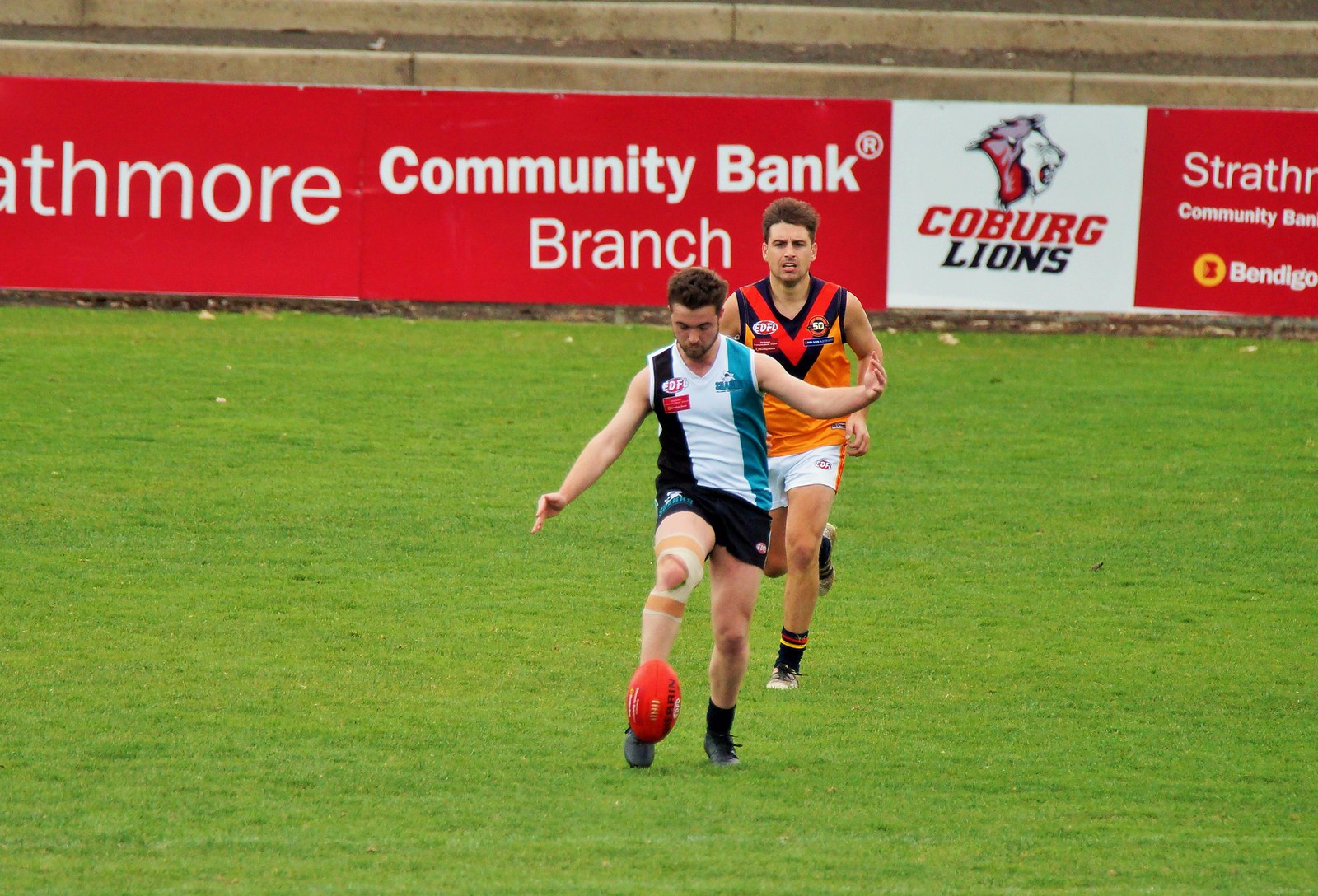In this vibrant photograph of an Australian rules football match, two men are captured mid-action on a lush green field. The man in the foreground, donning a black, white, and teal vertical striped jersey and black shorts, is about to kick the distinctly oval-shaped, bright orange football. His right knee is noticeably bandaged up, hinting at a possible previous injury. Behind him, an opponent in pursuit is clad in a striking uniform composed of white shorts and a jersey featuring bold colors of white, orange, black, and red forming a V-shape at the top. Both athletes are Caucasian. The backdrop of the image includes a variety of advertisements, prominently displaying "Community Bank Branch" and "Coburg Lions," suggesting this could be the home field of the Coburg Lions team, alongside other indistinguishable ads. The vivid colors and dynamic positioning of the players underscore the intensity and excitement of the moment.